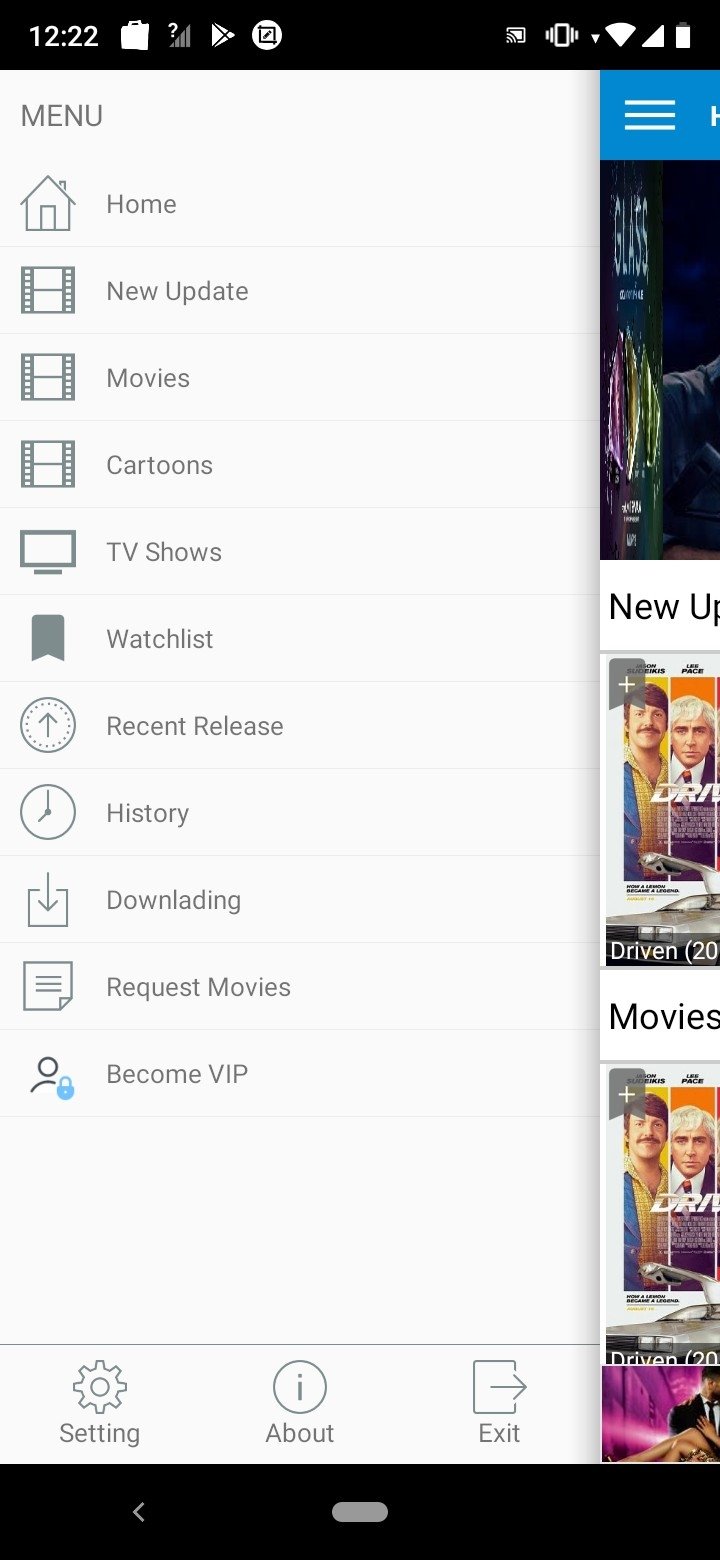In the screenshot captured from a smartphone, we view a detailed menu interface, which appears to be part of a media application. The layout is sophisticated, featuring an elegant off-white background. At the top, icons and labels are present, starting with a house symbol representing the Home menu. Adjacent to it, there is an icon resembling a piece of film on a reel labeled "New Update."

Below this, another film reel icon is labeled "Movies," followed by a similarly designed reel icon marked "Cartoons." A television icon signifies "TV Shows." Scrolling further down, the menu items continue with options such as "Watch List," "Recently Released," "History," "Downloading," "Request Movies," and "Become VIP," each neatly listed below a dividing gray line.

At the bottom of this section, additional options for "Settings," "About," and an "Exit" icon are displayed. The interface transitions to a black bar containing the text "New Update on Movies."

Below this segment, a collection of movies is shown in a three-column format. Although the labels on these movies are not legible, one movie prominently features two actors, with an executive producer credit at the bottom. Another highlighted movie showcases an image of a man carrying a woman against a peach-colored background. The overall design of the menu is organized and visually appealing, providing a clear and user-friendly navigation experience.